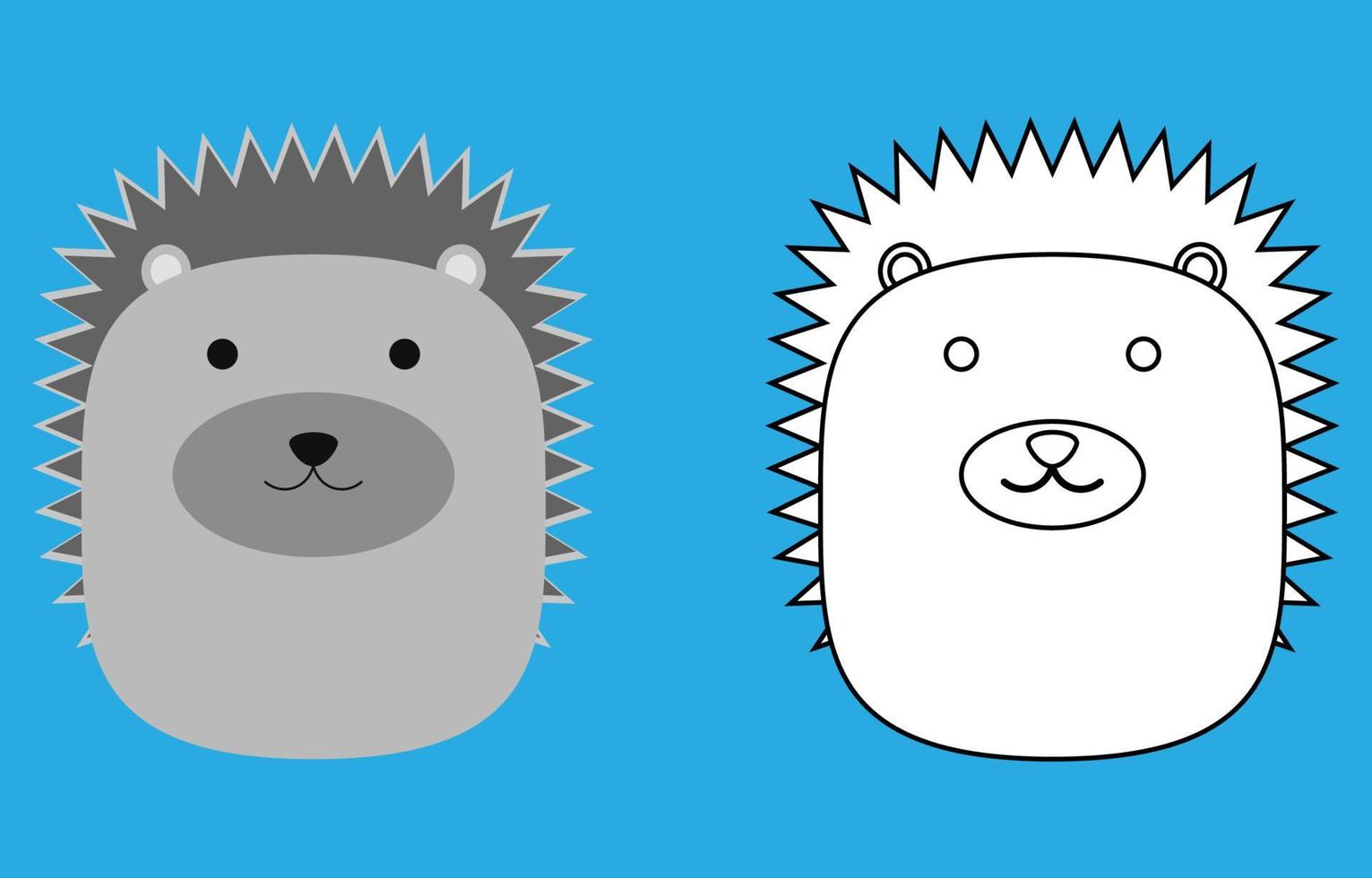The image features two side-by-side drawings set against a light sea blue background. On the left, there's a colored, complete drawing of a gray animal that closely resembles a hedgehog or a bear with spikes extending from its chin, over its head, and down its back. The creature has small, rounded ears, black dot eyes, a small black nose, and a simple line for a mouth. The body is primarily gray, with brown spikes adding detail. On the right, the same drawing is presented, but in black and white line art. The right-side line art version lacks coloring and portrays the same creature, with outlined features including circular eyes, a triangular nose with a smile beneath it, and the spiky outline around its body.